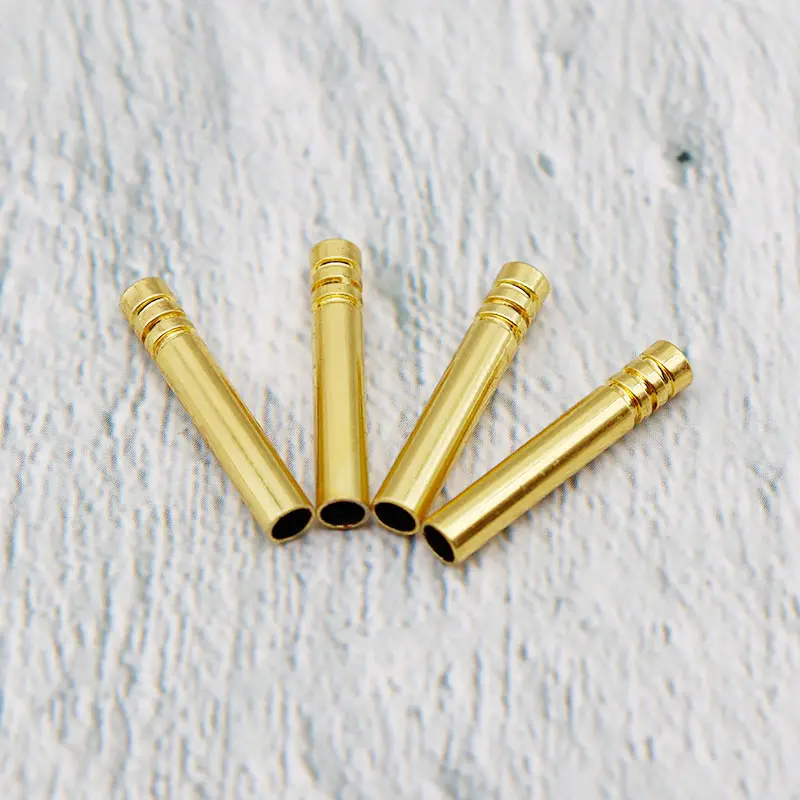This detailed color photograph features a close-up of four small, slender, and hollow metallic cylinders, arranged in a fanned-out pattern against a textured white surface. Each cylindrical tube, which appears to be made of gleaming, gold-colored metal, measures just a few inches in length. The tops of the tubes are intricately notched with three grooves, adding both aesthetic detail and ergonomic function to prevent slippage. The highly reflective, glossy finish of the cylinders suggests they could be custom caps, perhaps designed for the ends of shoelaces or pull-strings on clothing, though their exact purpose is not definitively known. The tubes' precise arrangement and polished appearance indicate a professionally staged product image, possibly computer-generated.